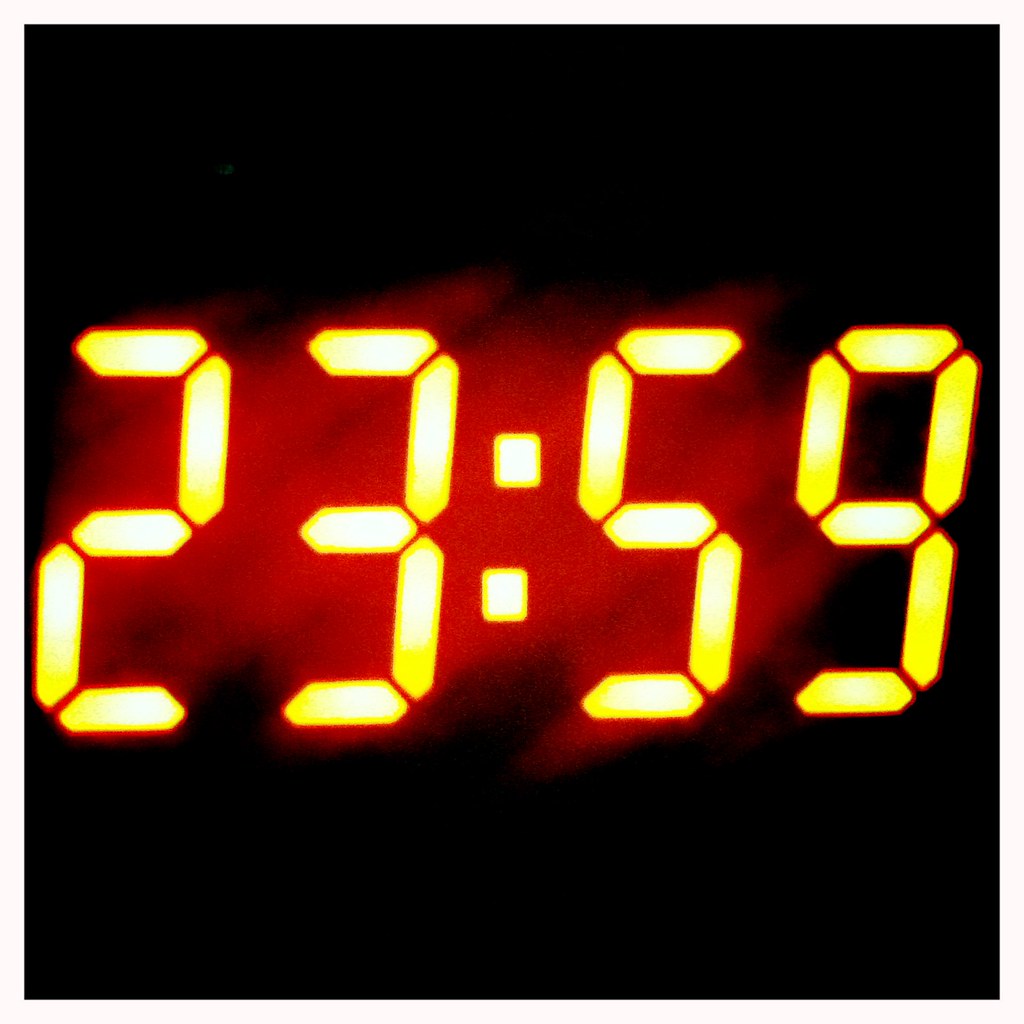The image is a close-up of a digital clock displaying the military time 23:59. The numbers are vividly illuminated in a bright gold-orange hue, casting a striking contrast against the predominantly black background. Positioned centrally, the numbers appear almost as glowing bubble-like segments. A semi-colon separates the 23 and 59, and around the digits is a distorted, oval-shaped red aura, which is brightest directly behind the numbers and fades into the darkness. This dramatic red smoke of light adds an eerie and intense atmosphere to the image, emphasizing the time displayed at the final minute of the day.